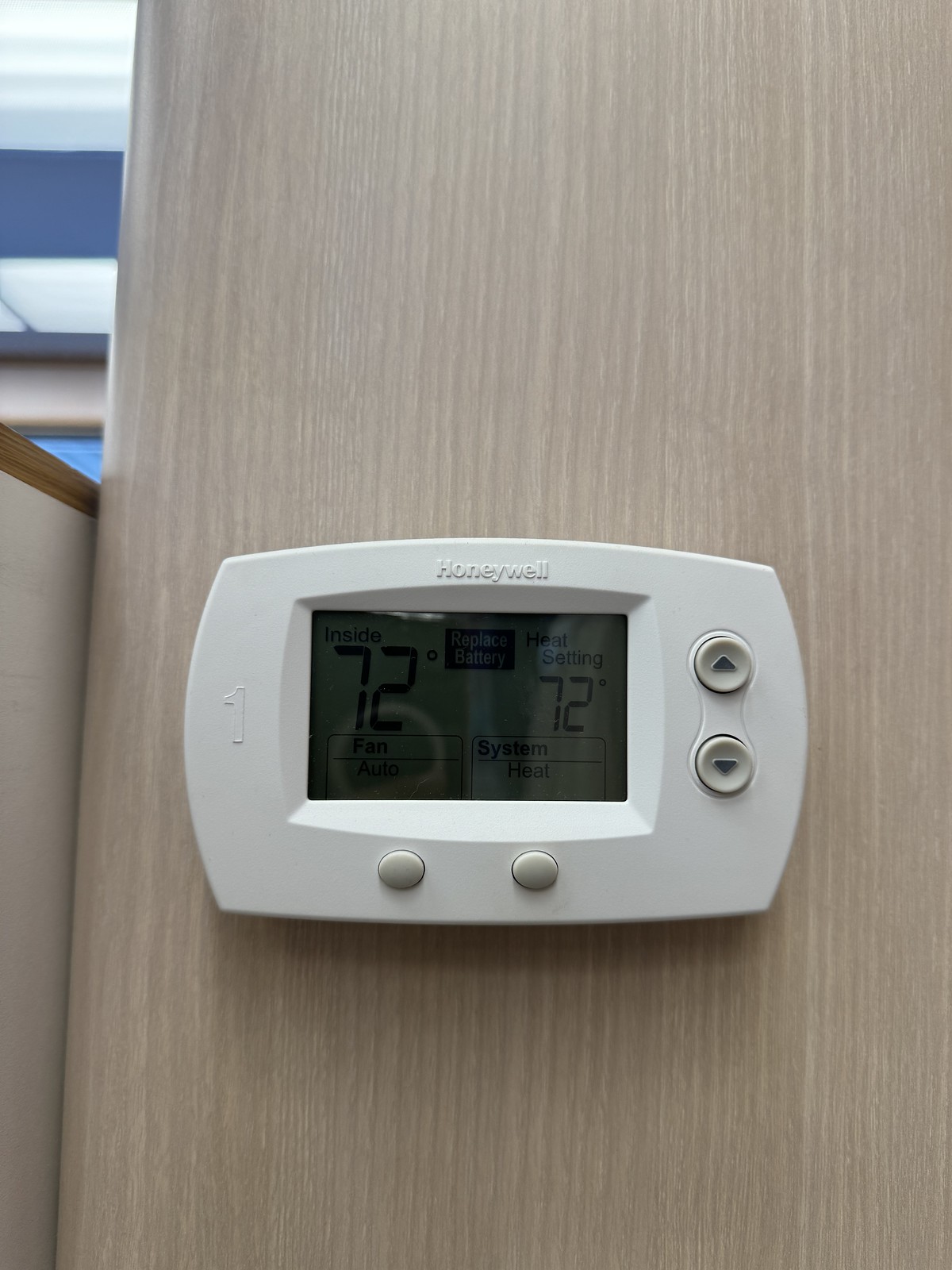The image captures a scene dominated by a wooden board with a varnish finish, occupying about 90-99% of the frame. The aspect ratio appears to be approximately 16:9. The photograph seems to be taken in an office space, hinted by the visible background on the left side. In the top-left corner, a light is faintly visible, illuminating part of the wooden surface. 

On the left side, a perpendicular white wooden board acts as a side frame for the main wooden board. The primary focus of the image is a Honeywell thermostat featuring a white frame. The thermostat displays the numeral "1" on its left side. On the right side of the thermostat, there are two arrow buttons for adjusting the temperature: one pointing up and the other down. Additionally, two gray buttons are positioned at the bottom of the device.

Notably, the thermostat's LED display is not lit up but still legible. It indicates that the inside temperature is 72 degrees Fahrenheit, with the heat setting also at 72 degrees. There is a flashing notification reading "replace batteries."